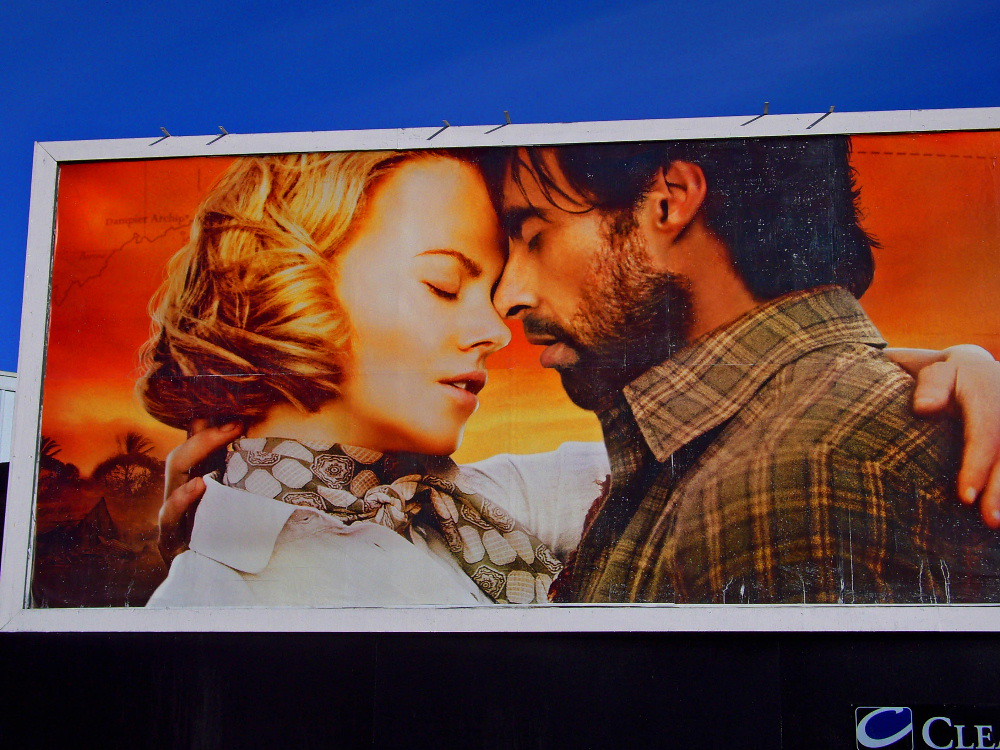This is a photograph of a large rectangular billboard framed in white. The main image features a tender moment between a man and a woman. The woman, positioned on the left, has short blonde curly hair and is wearing a white shirt with a scarf that appears to be brown with some white circles. Her eyes are closed as she leans in with her forehead touching the man's, their noses almost touching, and her mouth is slightly open. She has one arm around the man, her hand visible on his back, and she seems poised as if about to kiss him.

The man, positioned on the right, has dark hair, a dark beard, and mustache, and is wearing a green and yellow plaid button-up shirt. His eyes are also closed, and his mouth is slightly open. His hand rests on the back of her neck, adding to the intimacy of the scene.

The background of the image is a reddish-orange color, contributing to the warm tone of the photograph. Above the main picture, spanning horizontally, is a deep royal blue sky. In the bottom left corner of the billboard, there is a black square with a white outline and a white 'C' inside of it, next to the letters 'CLE' in white.